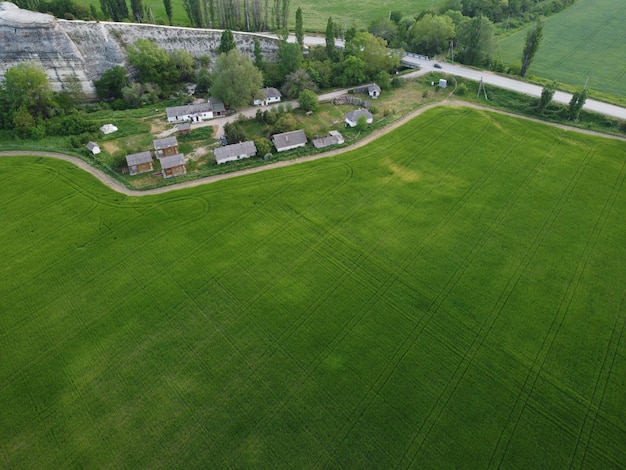This aerial photograph depicts a vibrant green landscape dominated by meticulously maintained fields, likely used for crops, marked with precise lawn patterns. In the forefront, the expansive field extends towards the middle, leading to a cluster of small houses and various buildings, all interspersed with patches of grass. A prominent road cuts through the scene from left to right, lined with trees and bordering the fields. On the far right, another road traces the edge of the terrain, ascending towards a jagged rock formation or cliff on the upper left. This rocky structure is gray and forms a striking contrast against the lush greenery. Surrounding this cliff base are trees and bushes, adding to the natural diversity. In the upper right section, additional fields and trees fill the view, creating a picturesque agricultural landscape.